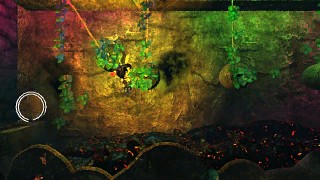The image depicts a point-and-click game set in an environment that strongly resembles a greenhouse or a cave-like structure. The background appears rocky, potentially the side of a vertical mountain or cliff, adorned with various colored lights—predominantly yellow, red, and green—casting an eerie glow. Some vegetation, possibly green vines, is seen hanging down from the upper sections. The image also displays a brick wall-like texture with patches of color: red on the upper left, yellow in the middle, and green on the right, resembling a painted surface. On the ground, there are speckled, round objects and what seems to be soil. A faint carpet-like element appears squished towards one side. A highlighted cursor on the left-hand side indicates the interactive nature of the scene. It's a compact, dimly lit visual, rich with layered details and interactive elements, amplifying the mysterious and exploratory ambiance typical of point-and-click games.